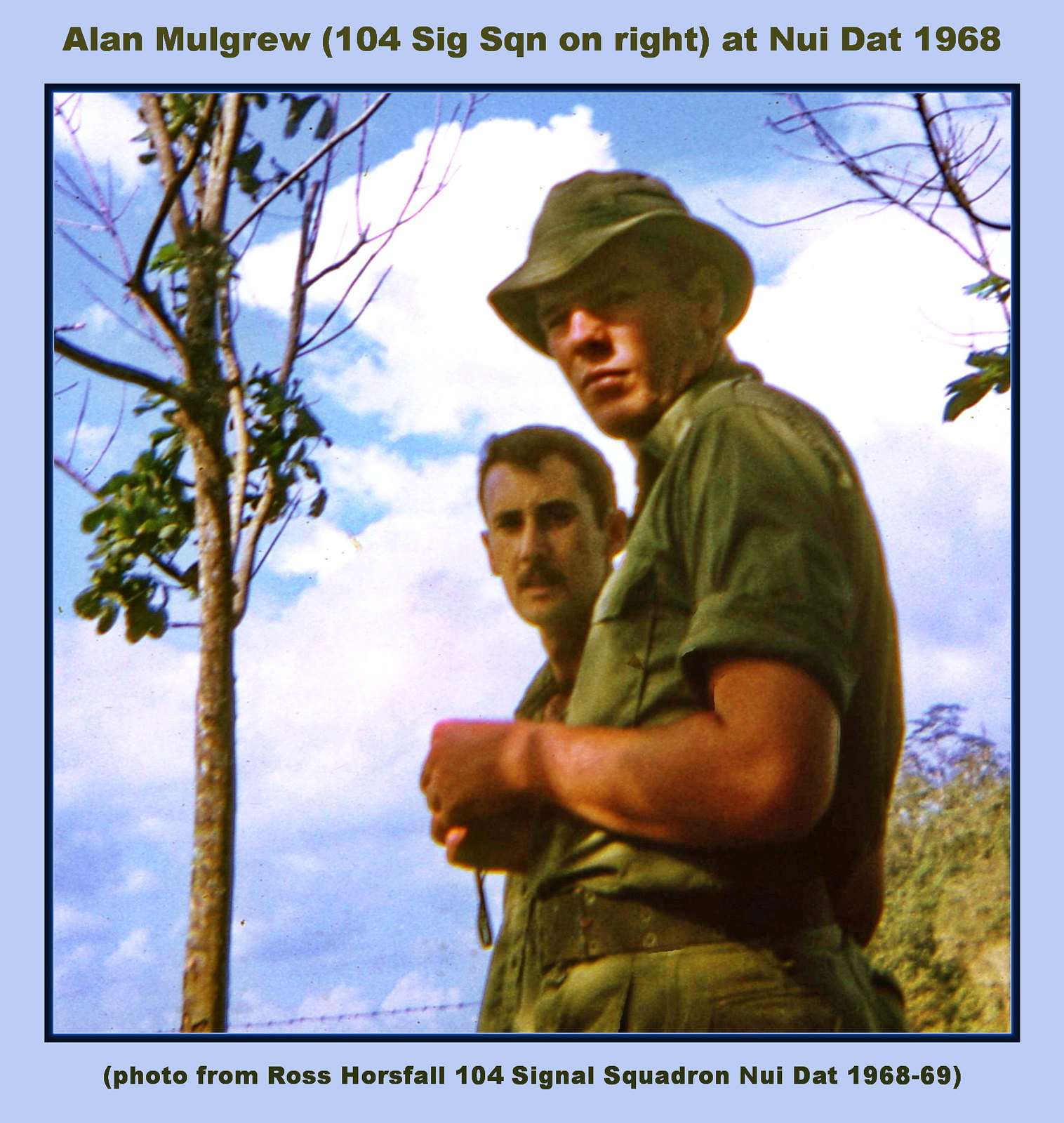This vintage photograph, set against a blue background with a thin dark blue border, features two men in military green uniforms at Nui Dat in 1968. The top of the photo is labeled "Alan Mulgrew, 104 Sig Sqn, on right, at Nui Dat, 1968" in olive green font, while the bottom reads "photo from Ross Horsfall, 105 Sig Sqn, Nui Dat, 1968-69." The man on the right, Alan Mulgrew, wears a floppy green hat and gazes intently at the camera. Next to him, a man with brown hair and a mustache is partially visible, wearing a similar uniform. Both are framed by a partly cloudy blue sky and sparse trees, adding to the scene's warm, possibly springtime setting. The names and units suggest they are members of the 104 and 105 Signal Squadrons during the Vietnam War.